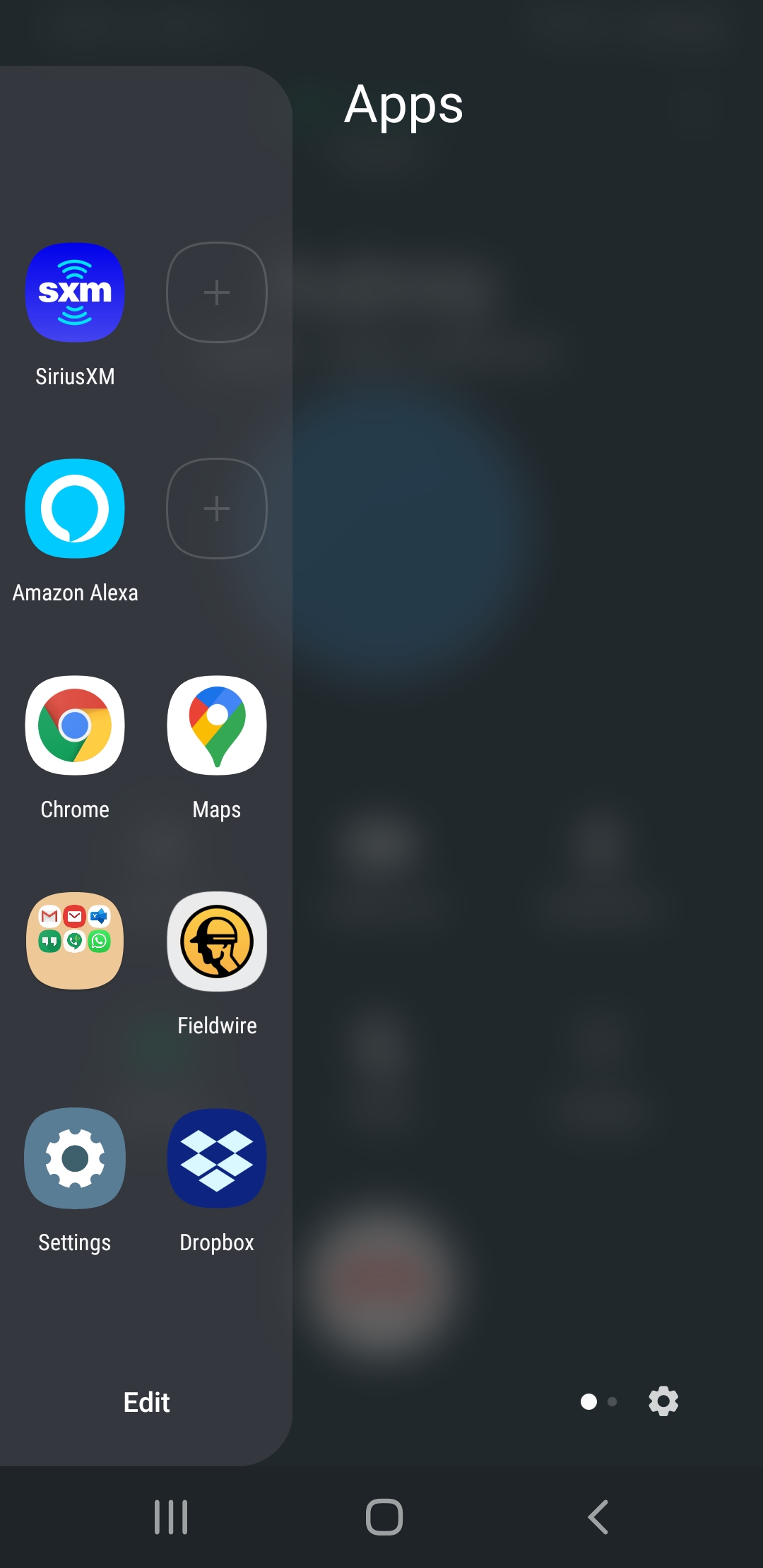This screenshot captures the display of an Android smartphone. At the bottom of the screen, you can see three on-screen navigation buttons: a triangle pointing left, a circle, and a square, indicative of the Android system, which contrasts with Apple's design that lacks these specific on-screen icons. Just above these navigation buttons, there are two dots, with the left dot bolded, indicating the presence of two home screens and that the current screen is the first. Adjacent to the dots is a gear icon, which likely leads to the device's settings menu.

The screen's upper segment features a white-font title, "Apps," overlaid on a standard metallic black background. The background, although slightly faded, suggests the presence of another layer beneath, hinting at an in-progress phone call with a contact, evidenced by a faintly discernible button at the bottom of the background.

Dominating the screen is an app panel that slides in from the left, displaying five rows of icons. In the top row, there's the SiriusXM app beside an empty spot. The second row contains the Amazon Alexa app next to another vacant slot. The third row features the Google Chrome and Google Maps apps. The fourth row appears to be a submenu, housing six apps, among which only Gmail and an app labeled FieldWire are recognizable. The fifth and final row includes the Settings app and Dropbox, with an "edit" option situated below this row, suggesting the ability to customize the app layout.

This detailed setup highlights the organization and functionality of the user's home screen, reflecting a blend of communication, navigation, and utility apps.